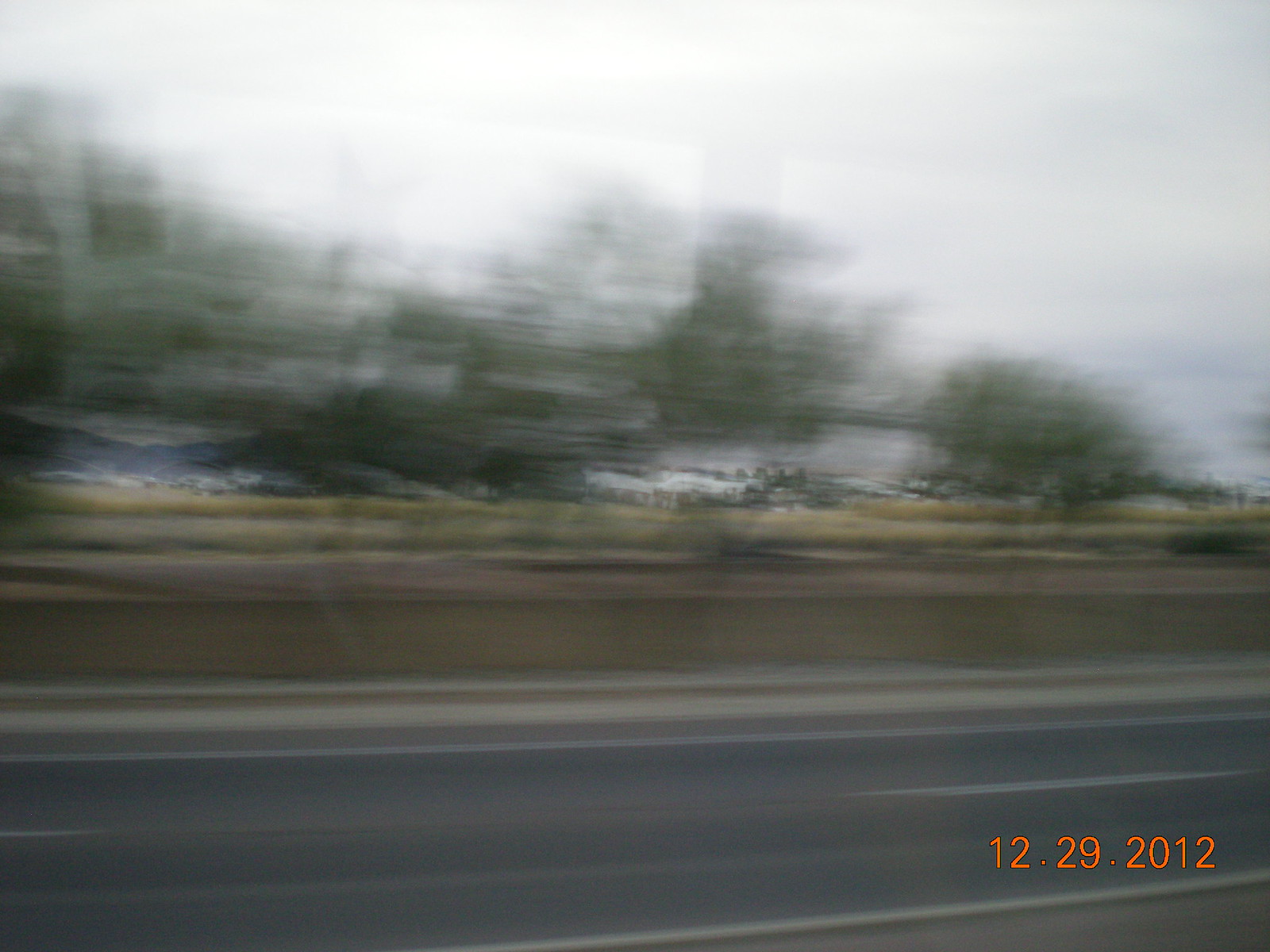This is a color photograph, though its extreme blurriness makes discerning details challenging. The image appears to be taken from the side of a road, possibly from a moving vehicle. The timestamp "12.29.2012" is overlaid in orange print at the bottom right corner. Distinctly visible at the bottom of the photo is a grey, blurred road, bordered by a pavement. Beyond this, there lies either a wall or a strip of green grass, alongside patches of lighter green grass further in the background. Above this, indistinct green masses suggest the presence of trees, their leaves rendered indistinguishable due to motion blur. Just below the tree line, the faint outlines of what might be buildings with white roofs are visible. The sky transitions from a whitish-grey on the left and center to a darker, bluish-grey towards the right side of the image.